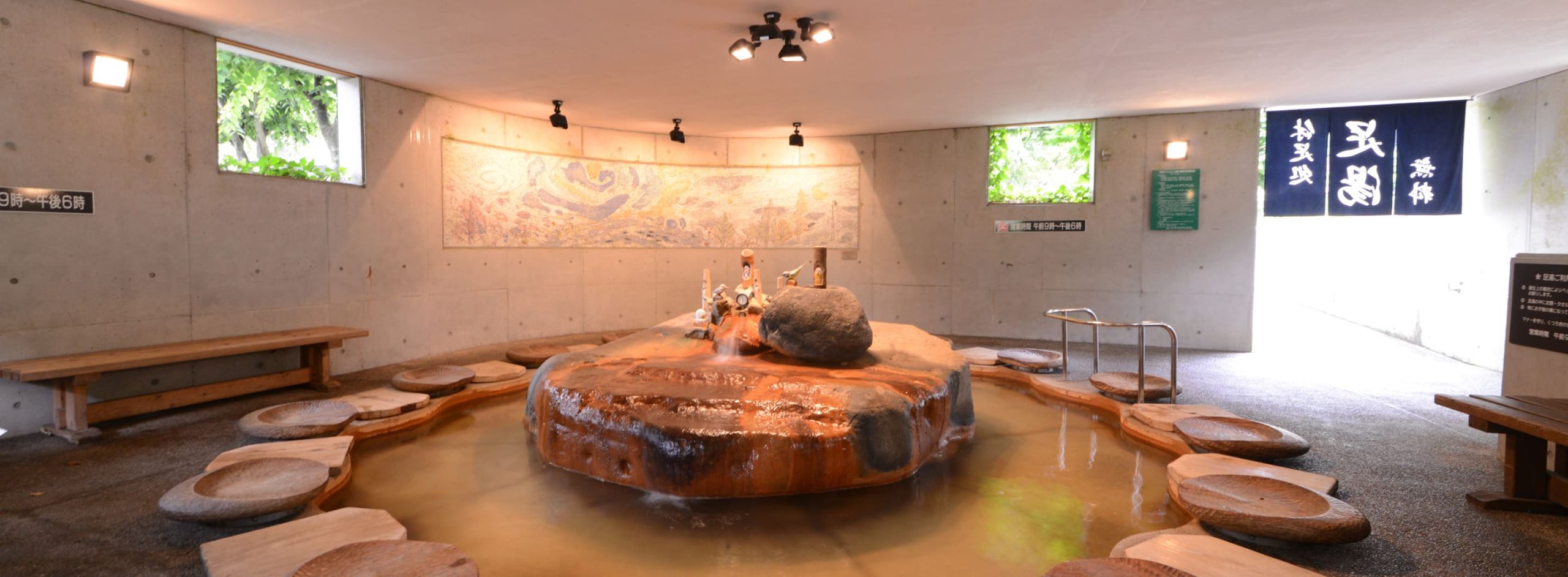This image depicts an inviting room in an upscale Asian spa designed for relaxation and therapeutic gatherings. The room’s focal point is a serene, shallow pool at the center, which houses a large, round stone that might function as a fountain. Surrounding this central feature are multiple round, wooden, bowl-shaped seats, each with a hollowed-out center, implying a seating area for at least ten people. To one side of the room, there are wooden benches capable of seating multiple individuals comfortably.

The room's design is characterized by its curved walls, featuring several windows that provide views of lush, green trees outside, letting in natural light. On the walls are various decorations; to the right, there's a long horizontal mural illuminated by three ceiling lights. Adjacent to this mural is a smaller window, beneath which hangs a long horizontal sign. Additionally, there's a striking blue painting adorned with Chinese characters and a large banner with oriental writing positioned in a hallway on the far right.

Overall, the tranquil environment, mixture of natural elements, and traditional Asian decor suggest a space dedicated to calming therapies, possibly including hot stone treatments, making it an ideal setting for relaxation and rejuvenation.